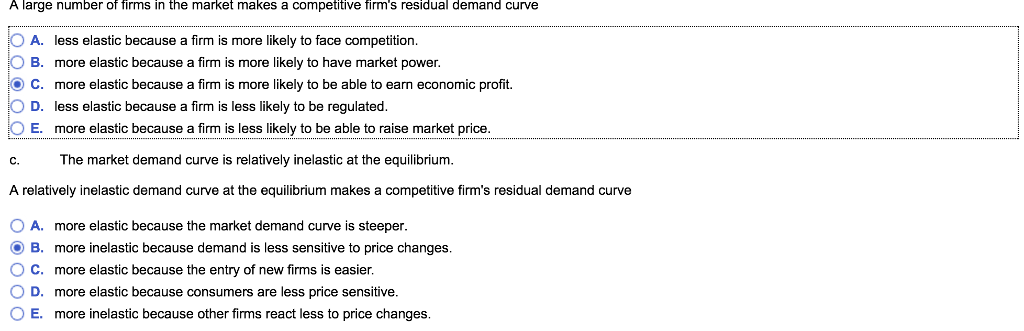In the image, there's a list featuring detailed explanations related to firms' market conditions. 

At the top left corner, the text reads: "A large number of firms in the market makes the competitive firm's residual demand curve." Directly below this statement, enclosed within a rectangular box, there are five letters—A, B, C, D, and E—each arranged vertically down the left side and colored dark blue. Adjacent to each letter on the left, there is a circle, with the circle beside the letter C filled in with dark blue.

Each letter corresponds to a specific description:
- Letter A is accompanied by the text: "Less elastic because a firm is more likely to face competition."
- Letter B states: "More elastic because a firm is more likely to have market power."
- Beside Letter C, the text reads: "More elastic because a firm is more likely to be able to earn economic profits."
- For Letter D, the description is: "Less elastic because a firm is less likely to be regulated."
- Finally, Letter E is explained with: "More elastic because a firm is less likely to be able to raise the market price."

Below these explanations, another question is presented: "A relatively inelastic demand curve at the equilibrium makes the competitive firm's residual demand curve."

The image diligently captures a comparison of different market conditions and how they affect the elasticity of a firm's demand curve.